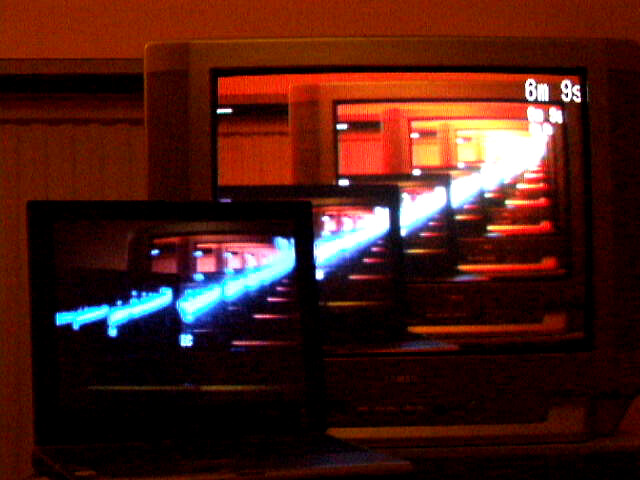The image depicts a surreal, almost infinite scene featuring two old televisions against a dark, reddish-hued background. At the forefront is a smaller TV, mostly black, displaying an image of the larger TV behind it, which has a grayish tint and a blurry label that might read "Samsung." Both TVs exhibit a series of interwoven white and blue lines that create a recursive, tunnel-like effect as if each TV is showing a scene of the other, continuing infinitely. The entire composition resembles a mirrored reflection that extends endlessly, reminiscent of looking into a line of mirrors. The background appears to be adorned with a dark red shading, and there is a timestamp in the corner reading '8m 9s'. The setting is framed against a brown wall, enhancing the vintage feel of the artwork.